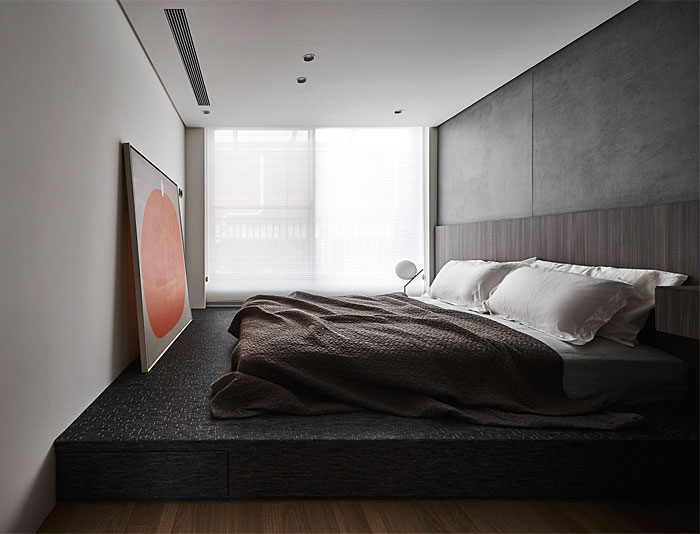This photograph captures a detailed scene of a contemporary bedroom, which likely resembles a hotel room situated within a city apartment. Dominating the room is a large, king-size bed with dark sheets and white pillows, positioned on an elevated black platform without a traditional bed frame. The bed, which appears to have been slept in and hastily covered, sits against a charcoal gray wall adorned with a sophisticated dark wood headboard. In contrast, the other walls and ceiling are pristine white, lending a crisp aesthetic to the space.

To the right of the bed, a sizable window offers a view of a neighboring building across the street, hinting at the urban environment. Leaning against the same gray wall behind the bed is a striking piece of art: a white canvas emblazoned with a vivid red or orange circle, accentuating the modern decor. Additional details include a brown blanket draped over the bed, recessed lights in the ceiling, a vent, and brown wooden flooring, all contributing to the room’s contemporary and slightly disordered charm.